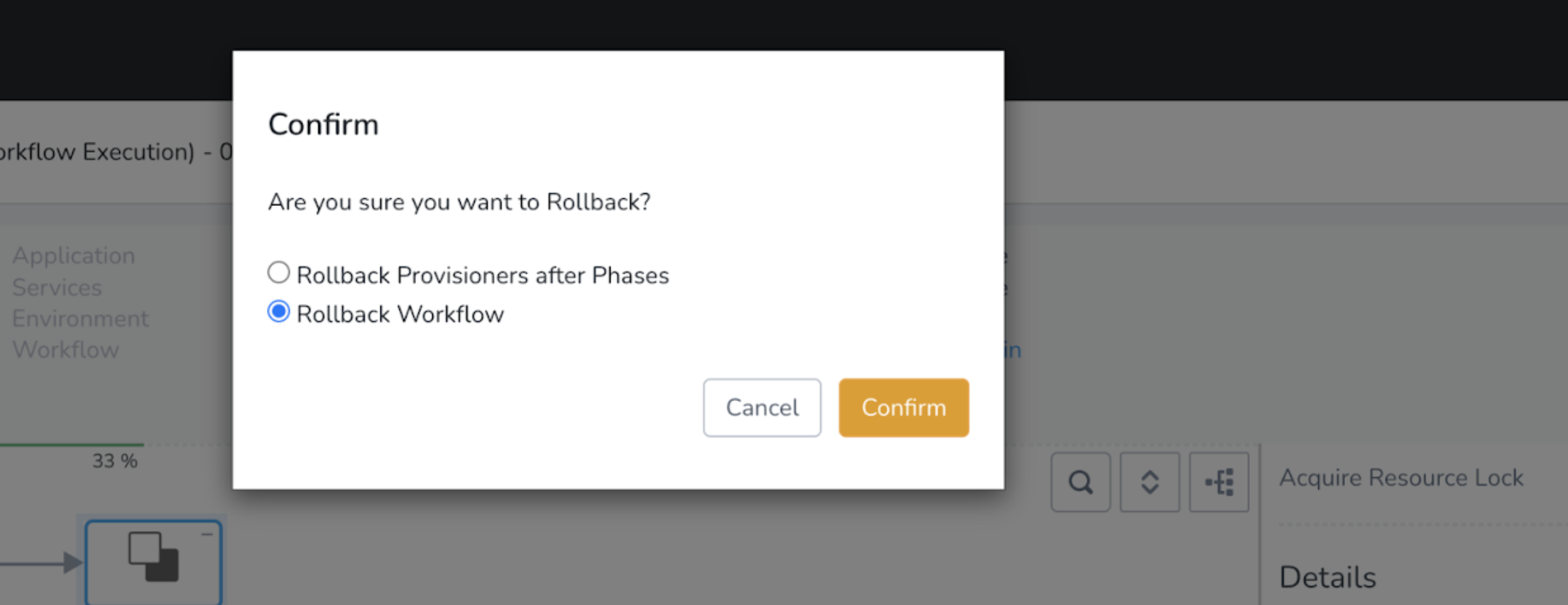The image depicts a detailed web page interface. At the top of the page, a black border spans horizontally, just below which the text "Workflow Execution" is prominently displayed. The left-hand column is organized with the labels "Application," "Services," "Environment," and "Workflow". Underneath these sections, a green horizontal line is visible, followed by the percentage "33%". An arrow pointing to the right nearly touches a blue-bordered square, which contains two overlapping squares— the bottom one is black while the top one is white with a black border.

In the bottom right corner of the page, the text "Acquire Resource Lock" is displayed above the word "Details". Overlapping this entire content is a pop-up window with a white background, prominently featuring the bold text "Confirm". Below this header, the message "Are You Sure You Want to Roll Back?" is displayed. Two radio button options are presented: the first, unselected option, reads "Roll Back Provisioners After Phases", while the second, selected option reads "Roll Back Workflow", indicated by a blue-filled circle. At the bottom of the pop-up, there are two rectangular buttons – a gray button labeled "Cancel" and an orange button labeled "Confirm".